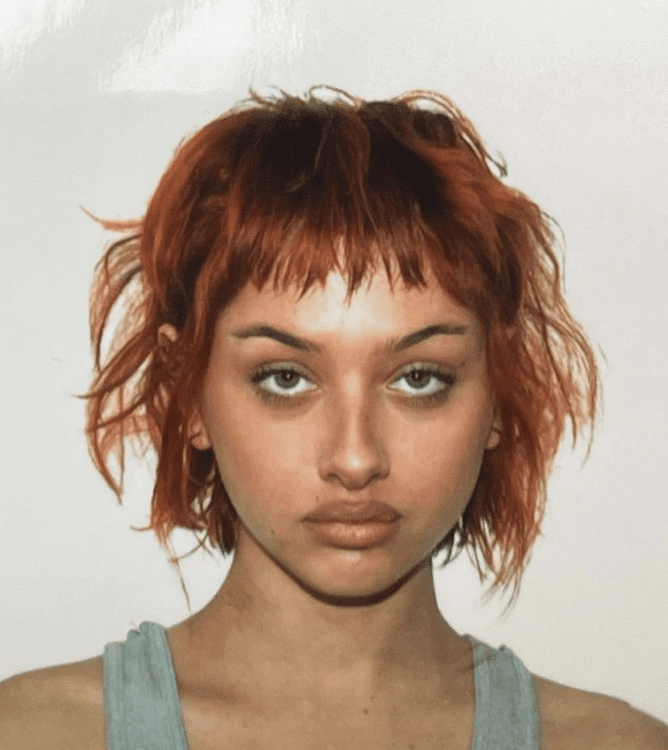This is a close-up photograph of a young woman with intentionally disheveled auburn hair that falls just below the middle of her neck. She has bangs that lightly touch her forehead and slightly obscure her straight, brown eyebrows. Her eyes are a deep brown, and she gazes directly at the camera with a serious, almost expressionless look on her face, revealing no hint of a smile. Her skin is olive-toned, and a subtle glare from the light reflects off her forehead. She is dressed in a gray tank top, the thin straps of which are visible over her shoulders. The background is a very light gray, almost white, emphasizing the woman’s features and her stoic demeanor. Her ears are partially visible, with her right ear more exposed than her left.